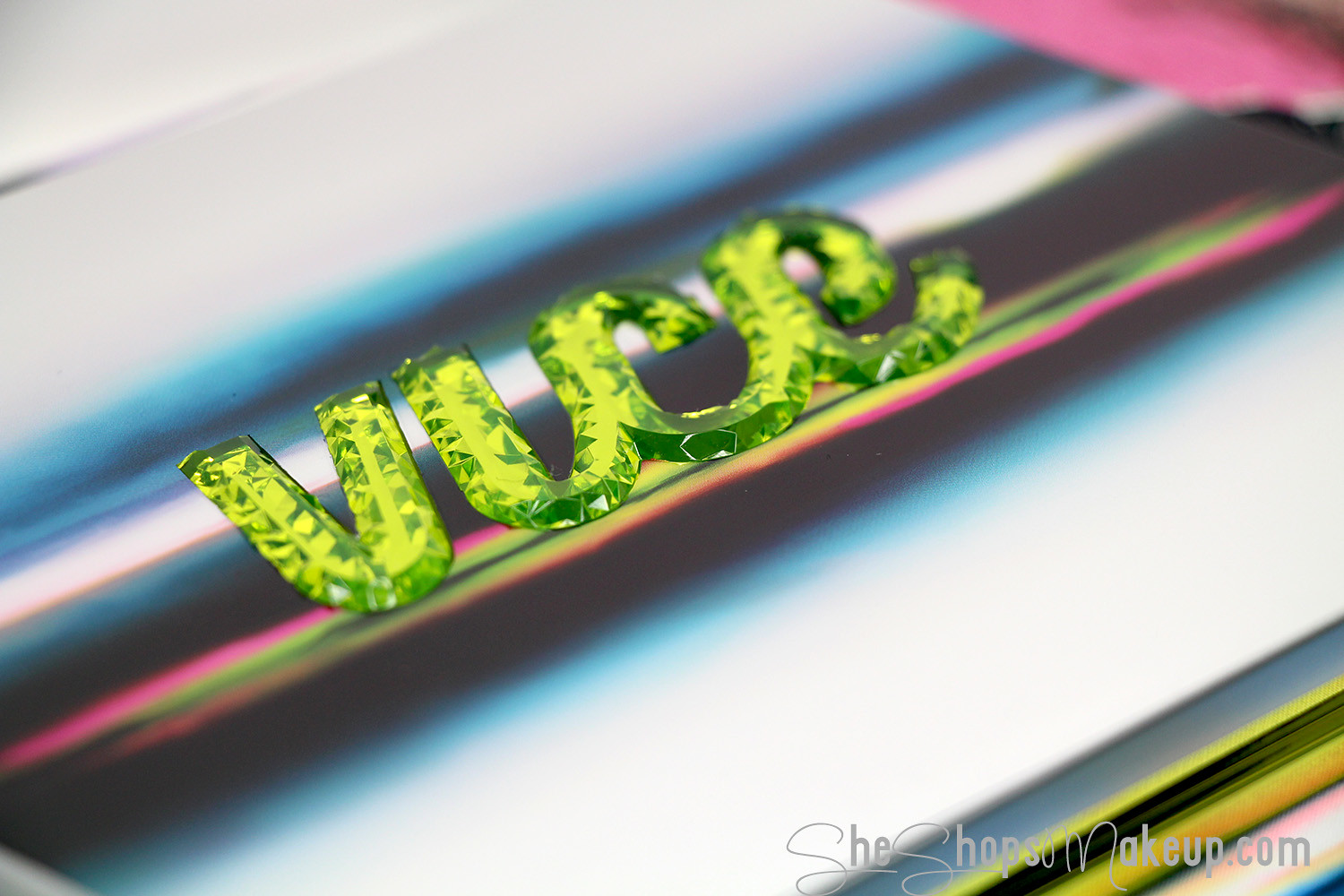The image features the word "VICE" displayed in a 3D cursive font that appears to be made from a transparent, gem-like material, possibly reflective glass or plastic, which creates a shadowy and gleaming effect. These letters are diagonally placed on a background consisting of blurred, colorful horizontal lines that include hues of blue, black, pink, green, and white, giving an impression of depth. The surface is somewhat indiscernible and abstract, with the colors and streaks artistically spliced together, enhancing the visual complexity. In the bottom right corner of the image, there is a gray watermark that reads SheShopsMakeup.com.